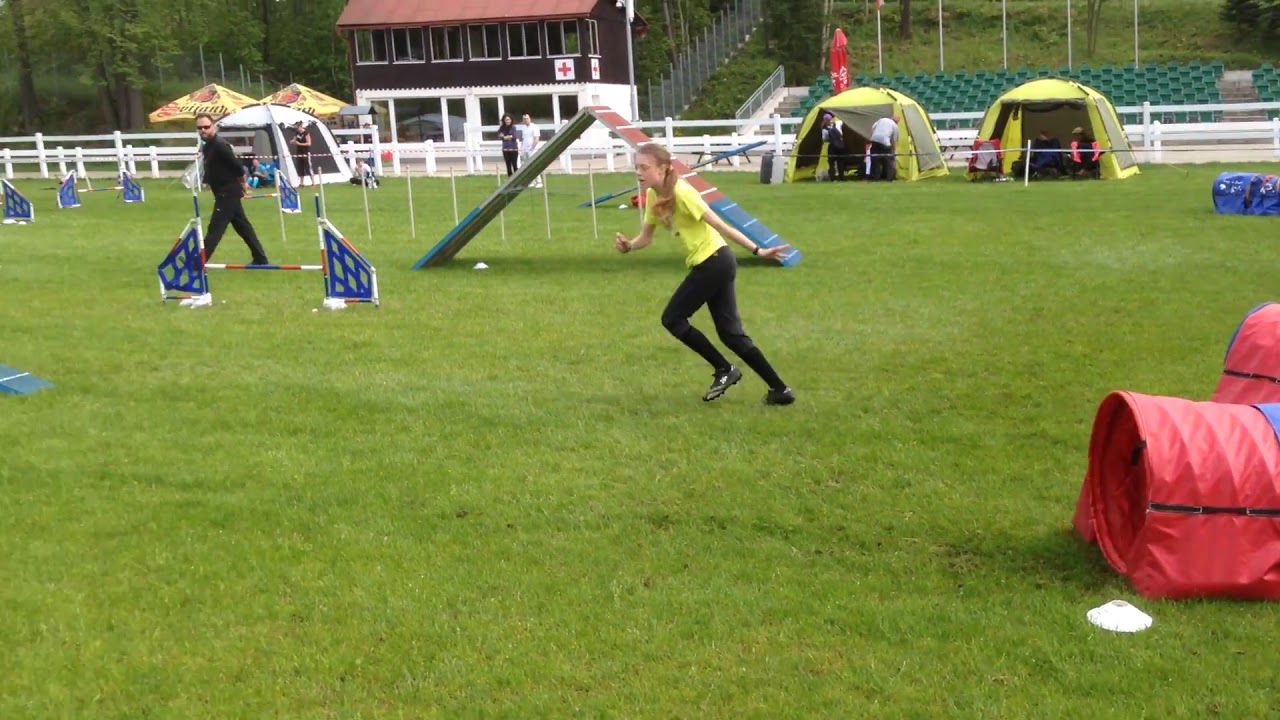The photograph captures an expansive outdoor field covered in vibrant green grass. In the foreground, a girl dressed in a bright yellow short-sleeved t-shirt, black pants, long dark socks, and grey-colored cleats with studs is captured mid-stride. Her long, orangeish-blonde hair is tied back into a ponytail that extends past her chest. She's positioned amidst a variety of training obstacles, seemingly engaged in a workout or warm-up activity. These obstacles, reminiscent of a dog agility course, include a small red and blue tunnel, yellow poles for jumping over, and a wooden ramp set up like the top part of an A-frame.

A man wearing a black shirt, black pants, and dark sunglasses stands nearby, closely observing the girl's progress, likely her coach or trainer. In the background, there are yellow tents set up near the field boundary, which may house spectators or parents. Beyond the field, a brown and white building displaying a hospital symbol is visible, with green trees towering above. Additional features include bleachers with green chairs, a white fence, and what appears to be a concession or first aid stand beneath umbrellas, adding context to the busy yet orderly setup of this vibrant outdoor scene.